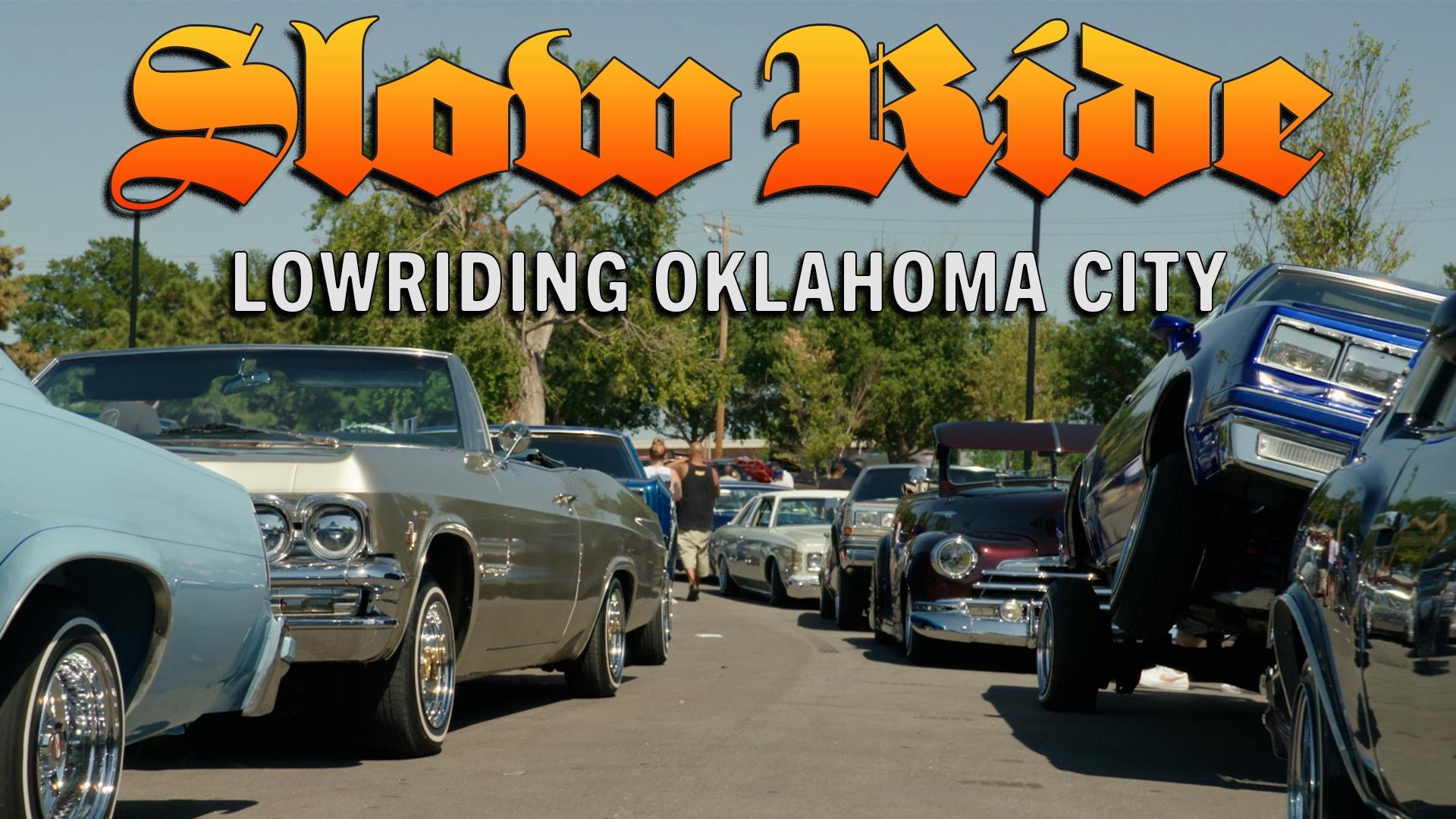The flyer advertises a car show event specifically for slow riders in Oklahoma City, titled "Slow Ride, Low Riding Oklahoma City." The text "Slow Ride" is displayed in prominent, fancy, 3D-style block letters with a yellow to orange gradient, while "Low Riding Oklahoma City" is in skinnier, white block letters, also with a 3D effect. The poster features rows of vintage low rider hot rods, known for their customized hydraulics that allow them to bounce along the street. One of the showcased cars is dramatically tilted on its hydraulics. The event setting appears to be a street scene with shiny, well-maintained classic cars, including a gray car facing the viewer and a blue car with its rear end lifted, showcasing its undercarriage. The backdrop includes utility poles, large trees, and people walking among the cars, lending a lively atmosphere to the scene.